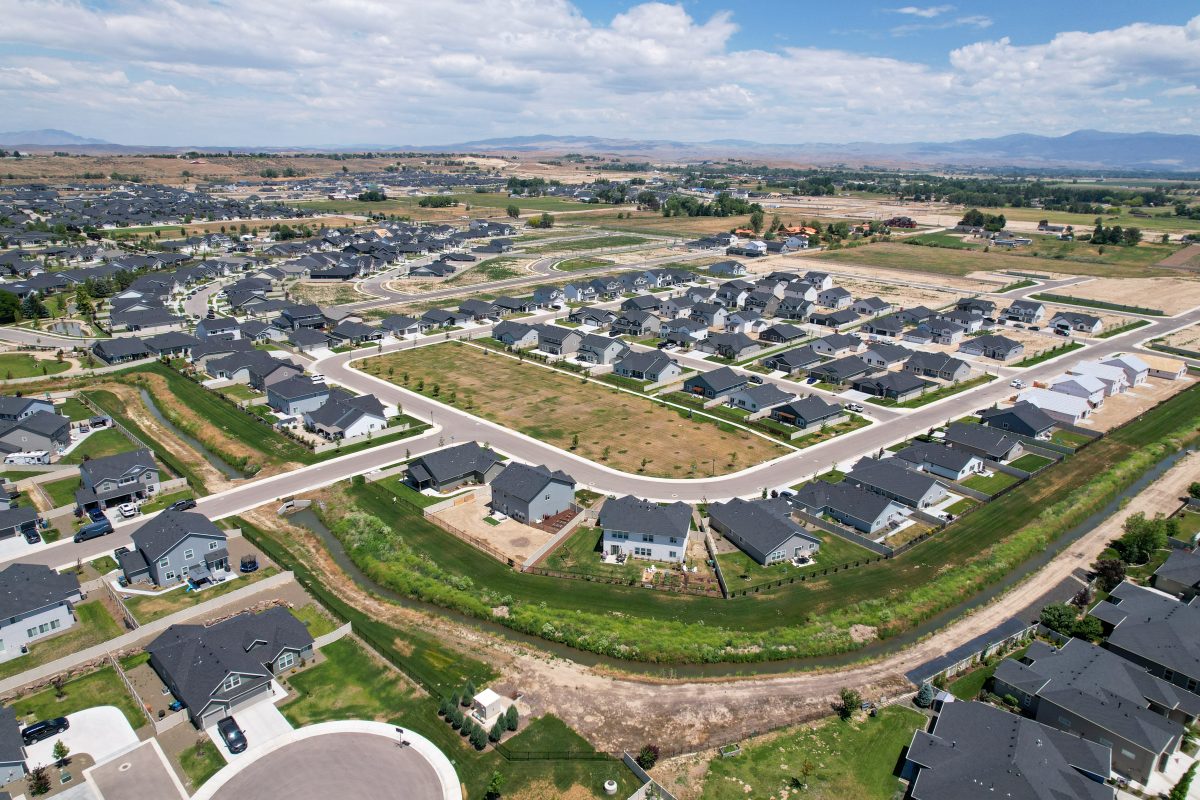This aerial view captures a modern housing development spread across flat terrain, characterized by its suburban layout and lack of mature vegetation, hinting at its relatively new establishment. The majority of the houses, predominantly one-story with a few two-story structures, feature gray or dark gray roofs with light gray or white exteriors. The central roadway is U-shaped, flanked by homes oriented horizontally between the parallel roads and others lining the exterior. An intersecting road towards the center-left divides additional clusters of similar houses. In the foreground, a circular turnaround marks the end of a feeder road leading into the neighborhood, while a stream meanders through or around the bottom of the image. Sparse greenery punctuates the scene, with dirt patches indicating a dry environment. The backdrop includes distant low mountains under a mostly cloudy sky with a dark blue hue in the upper right, signifying good lighting on what appears to be a sunny day. The entire development extends until it meets the horizon, blending housing and nature.